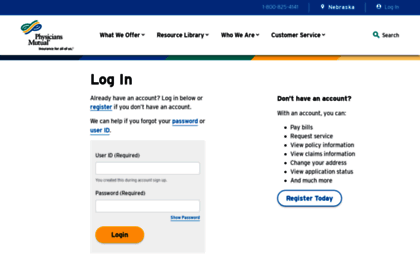Screenshot of a website or app interface, featuring a minimalist design with a predominantly white background. The uppermost section displays a blue text box on the right side containing a "1-800" number, a label "Nebraska" alongside a small dark location icon, and a "login" link. Below this, a navigation bar includes buttons labeled "What We Offer," "Resource Library," "Who We Are," and "Customer Service." A search box is also situated on the right side of this bar.

On the left side of the interface, the text "Physicians Mutual" is shown next to a logo with green, yellow, and blue colors. Below this logo, a rainbow-colored border adds a touch of vibrancy to the otherwise simple design.

In the main section, there are two centered columns. The left column features a login box where users can enter their User ID and password, accompanied by a login button. The right column includes a "Don't have an account?" section, which lists the benefits of registering in bullet points. At the bottom of this section, there is a prompt "Register Today" encouraging new users to sign up.